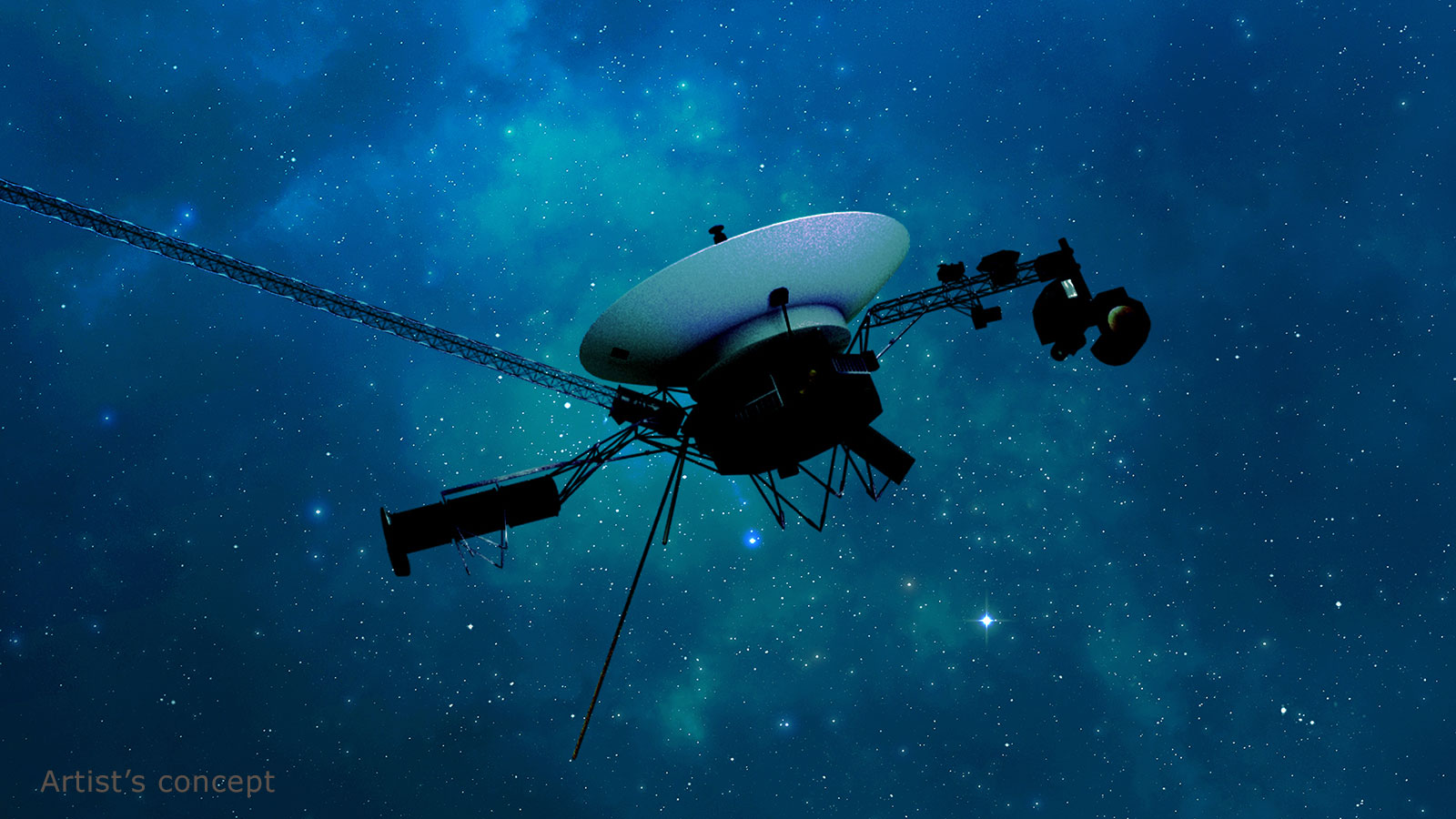The image depicts an artist's concept of a satellite floating in outer space. Dominating the scene is a white, dish-shaped component with a black piece at its center, its wide end facing upwards. This satellite features multiple black platforms and antennas extending from its sides. A chain-like structure stretches from the left side of the image, connecting to the device. The surrounding sky transitions from a deep, dark blue near the edges to a lighter blue towards the center, accented by an array of twinkling stars and a few glowing, neon-blue dots. Among the stars, a notable cluster shines brightly with blue and purple hues, creating a vibrant backdrop for the satellite. The bottom left corner of the image is labeled "artist concept," confirming its illustrative nature.